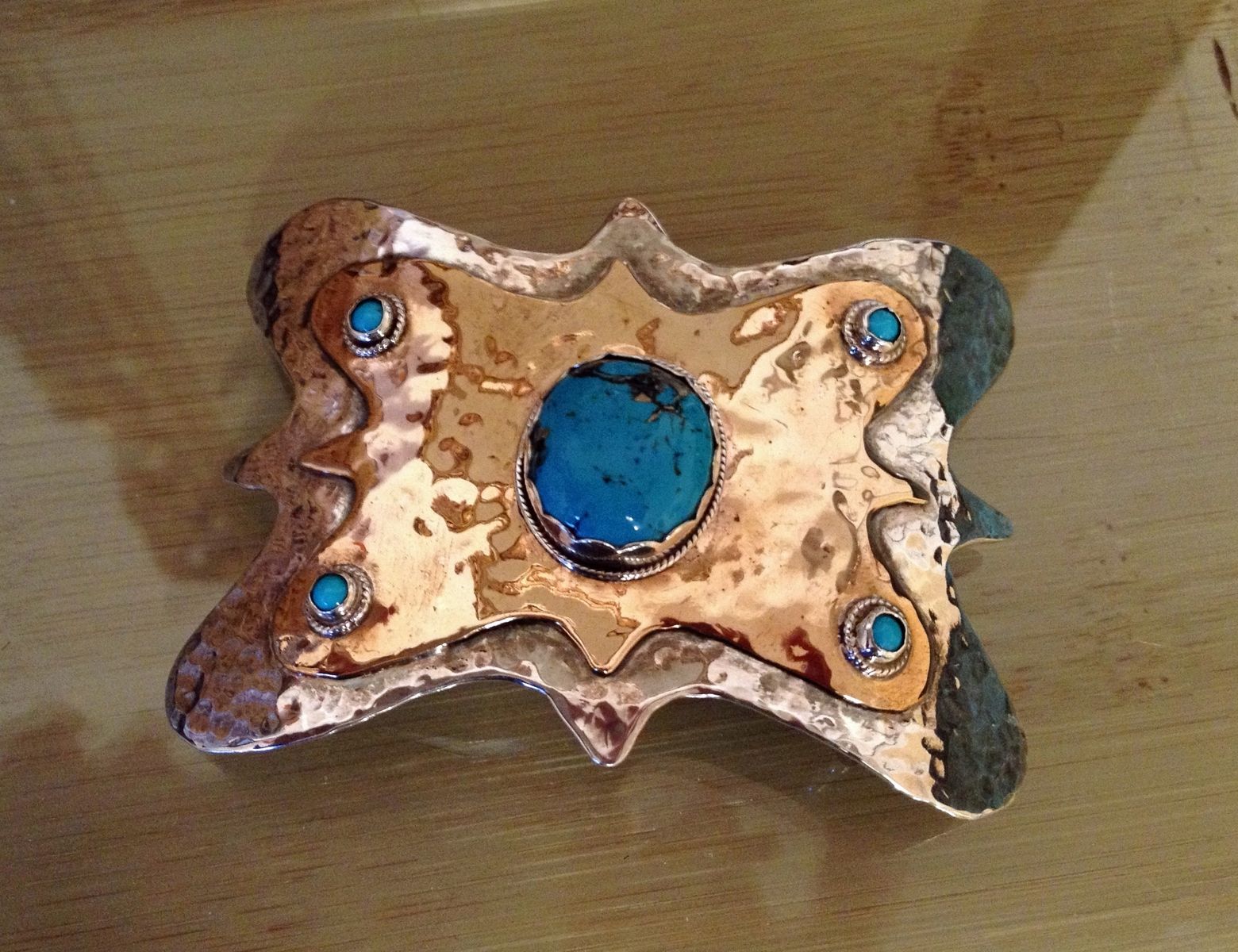The image depicts an intricately designed piece of jewelry, possibly a belt buckle, brooch, or decorative accessory for a bolero tie. It features a prominent butterfly-inspired design, though not a literal butterfly. The piece is crafted from a mix of shiny copper and silver-colored metals, with a textured yet glossy finish. Central to the design is a large, vibrant turquoise stone with brown striations, encased in a chrome or silver border. This main stone is surrounded by four smaller turquoise gems, one affixed to each corner of a lighter bronze or gold-hued attachment, each encased in silver. The jewelry is showcased on a shiny wooden table, accentuating its detailed craftsmanship and vibrant blue hues.